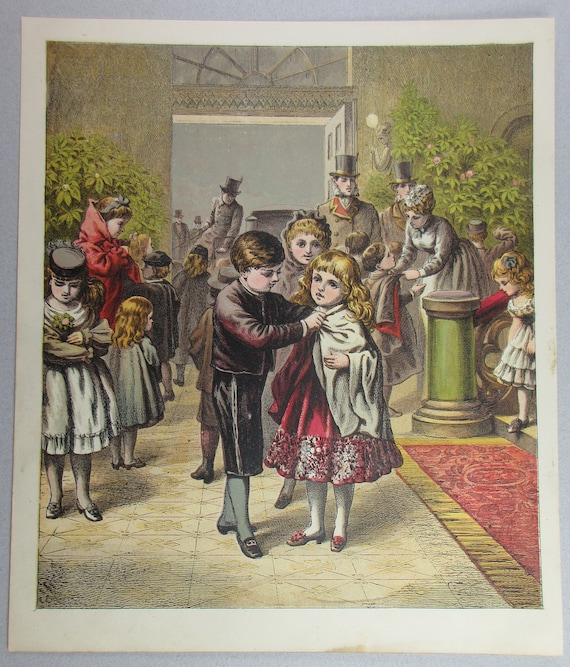A detailed 19th-century lithograph or etching depicts a luxurious Victorian interior bustling with children and adults. The room exudes opulence with its red and gold carpet, intricate furniture, and richly adorned walls. The predominant colors are shades of pale green, gray, pale red, and gold.

At the center of the image, a young boy with dark brown hair, dressed in a dark coat, knee-high shorts, gray tights, and black shoes with silver buckles, is assisting a blonde girl. The girl, sporting rosy cheeks and bangs, wears a vibrant red dress adorned with fancy hem patterns, white tights, and beige shoes with red bows. The boy is fastening a white cloak on her that reveals a red lining inside.

To their left stands another blonde girl in a greenish-blue coat, white tights, and black shoes. Behind her, a slightly older girl with yellow hair, a round black hat, and a white dress decorated with a green flower with pink in the middle gazes at the scene. A woman behind them, cloaked in a red shawl reminiscent of Little Red Riding Hood, surveys the room while another child, possibly a small boy, rummages through her shawl.

Further back, a woman bends to help a child with a black and red cloak, possibly preparing them for an outdoor excursion. Two men, distinguished by their black top hats with gold rings, oversee the proceedings. Adjacent to these scenes, a child with a white shawl covering her blond hair stands quietly, and another boy seems engaged with a green tree bearing pink flowers. Behind the foliage, a statue of a woman cradling a pole with a light enhances the Victorian décor.

In the rear, the room opens to an exterior where a coach driver in a top hat waits, perhaps to ferry the elegantly dressed attendees. The doorway offers a glimpse of another coach in the distance, adding a layer of anticipation and movement to the tableau. Matching the indoor grandeur, a stairway with a green column, red handrail, and another child in a white ruffled dress descending echoes the overall theme of refinement and elegance.